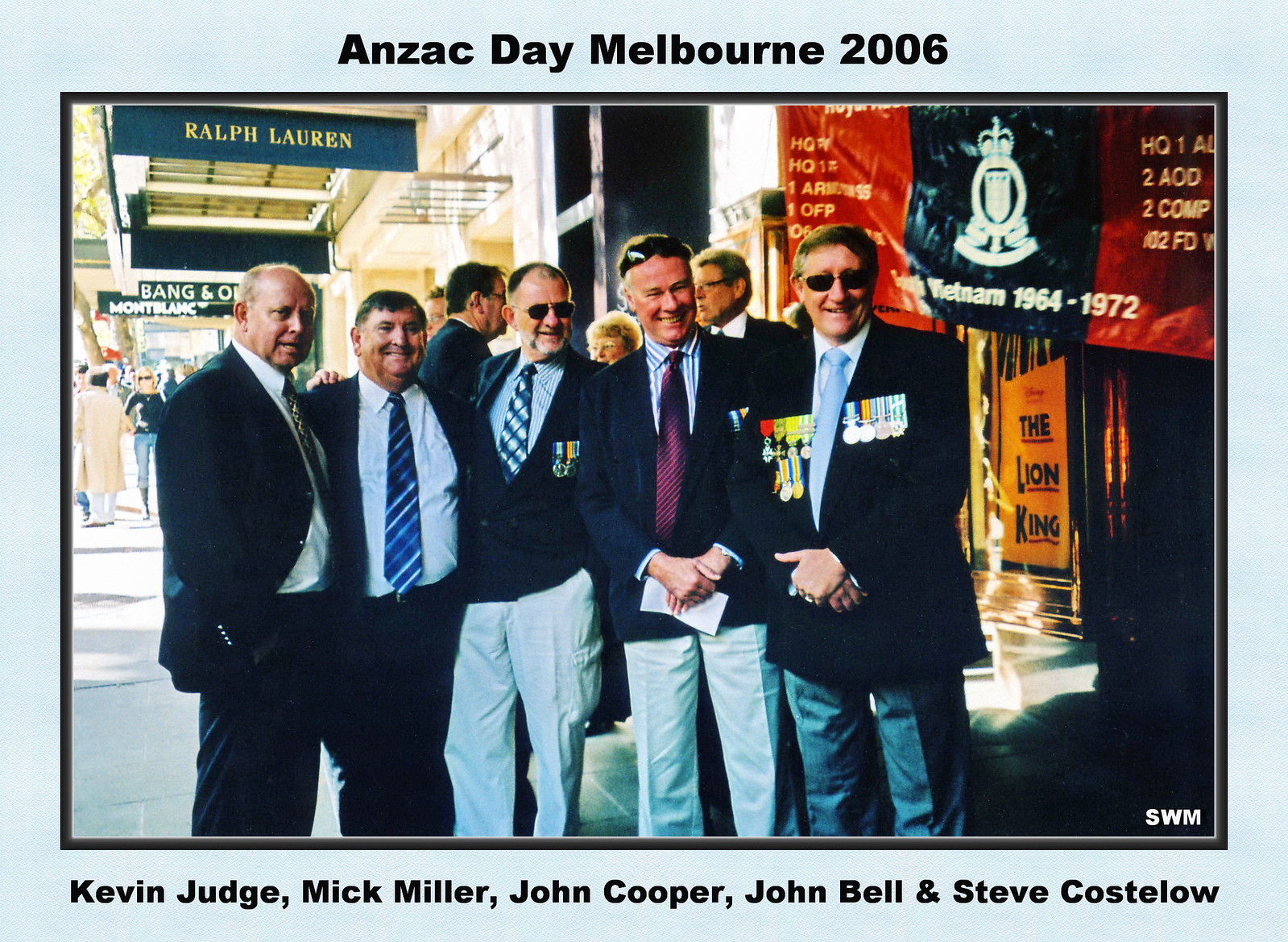The photograph, framed with a light blue border, prominently features five older white men standing side-by-side, posing for the camera. Text at the top of the image reads "ANZAC Day Melbourne 2006," while a caption at the bottom identifies the men as Kevin Judge, Mick Miller, John Cooper, John Bell, and Steve Costello. The men are dressed in black suit jackets paired with variously colored pants—two in black trousers, two in light-colored trousers, and one in dark gray trousers. Notably, three of the men on the right display military medals on their chests, with the man furthest to the right having the most medals. They are captured outdoors, in what appears to be a shopping plaza with visible store signs for Ralph Lauren and Mont Blanc. Additional background details include various banners, one of which references the Vietnam War (1964-1972). The setting is lively, with crowds and other people in the distance behind the men.